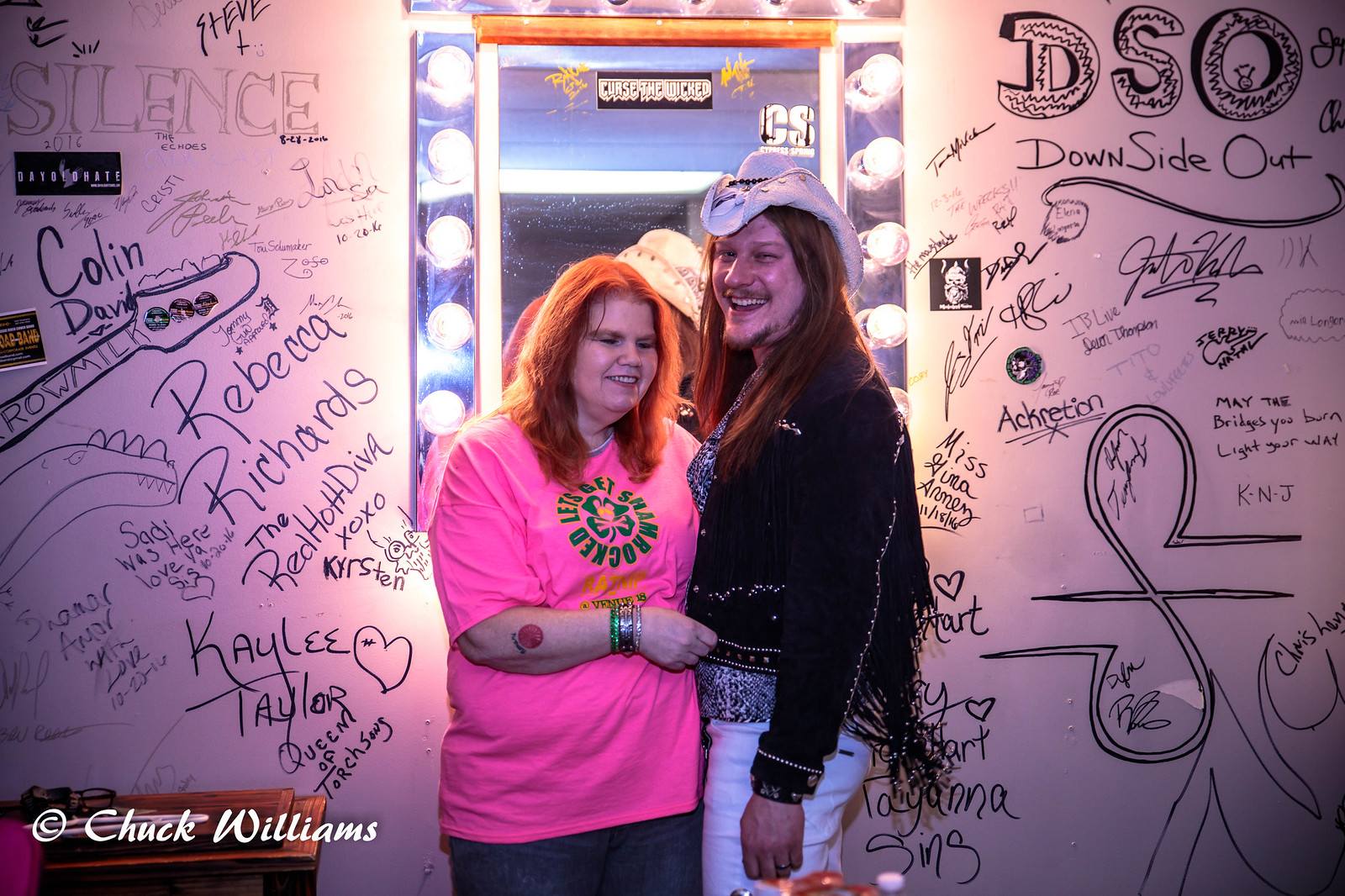The image is a rectangular backstage photograph capturing two people standing and posing together, half-embracing and smiling at the camera. The backdrop is a wall heavily decorated with autographs, band names, and graffiti, all done in black marker or pen. Notable inscriptions include "DSO, Downside Out," "Miss Xena," "Rebecca Richards, The Hot Diva," "Kaley Taylor," and "Plano Torch Song," along with various logos and symbols like a double S resembling a fishhook. Central to this wall is a vanity mirror bordered with lightbulbs, typically found in dressing rooms.

The young man in the photograph has long reddish hair, a black goatee and mustache, and wears a white cowboy hat. His attire includes a black country jacket adorned with fringe and sequins, a black and white snake print shirt, and white pants. The woman next to him has shoulder-length red hair and is dressed in a bright pink T-shirt. She sports a red and black tattoo on her forearm and sparkly bracelets on her wrist. Both individuals appear happy and content, with the woman posing cheerfully and the man looking amused. The bottom left corner of the photograph features the copyright sign and the name Chuck Williams, indicating the photographer.